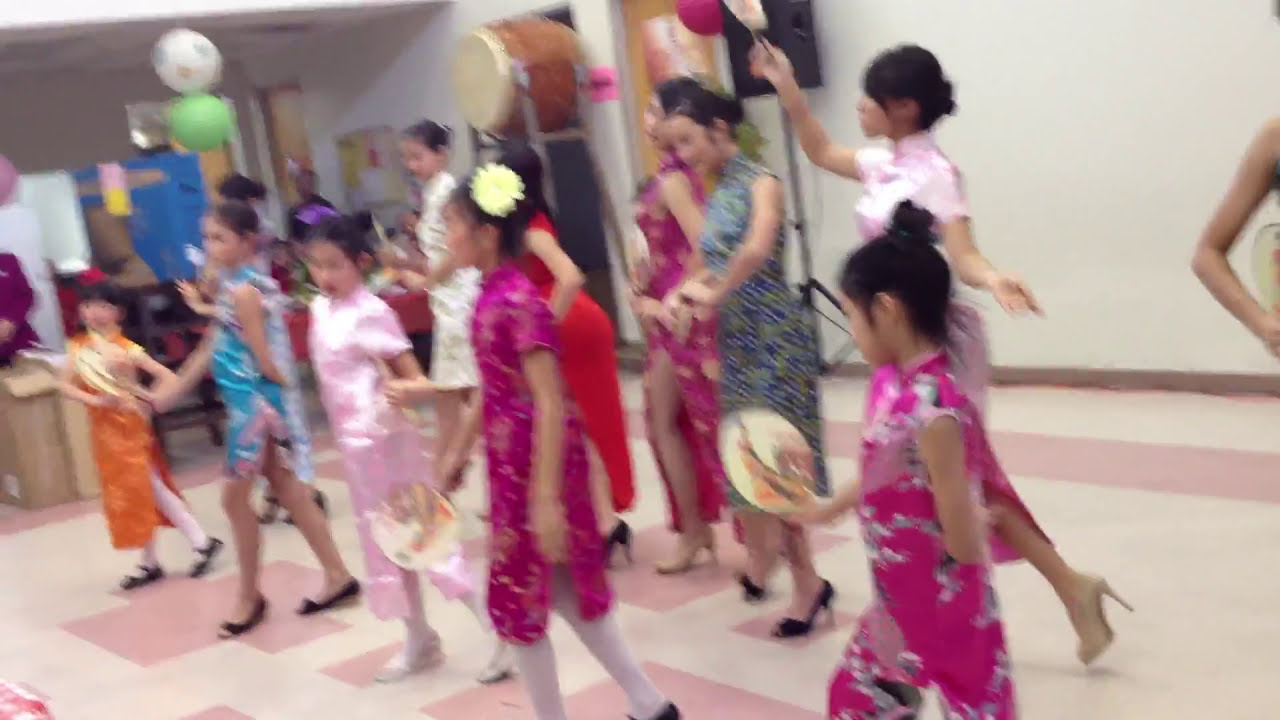The image captures a vibrant, indoor scene of young Asian women and girls performing a traditional dance. The room is brightly lit with white walls and a light tan floor adorned with pink tiles. The dancers, ten in total, form two rows and are facing diagonally towards the left side of the image. In the front row, there are five younger girls, aged approximately between 5 and 10 years old, dressed in colorful kimonos of hot pink, pale pink, blue, and orange, with shiny floral patterns. These girls wear black flats. The second girl from the right in the front row is notable for having a large yellow flower in her hair. Behind them stand the older girls, likely ranging from their teens to early twenties, adorned in similarly vivid kimonos and wearing heels. All the dancers have their black hair styled in buns. Adding to the festive atmosphere, there are green and white balloons visible in the top left corner. The image, although blurry due to the movement of the dancers, captures the energy and cultural richness of the performance, possibly taking place in a school gym or cafeteria.